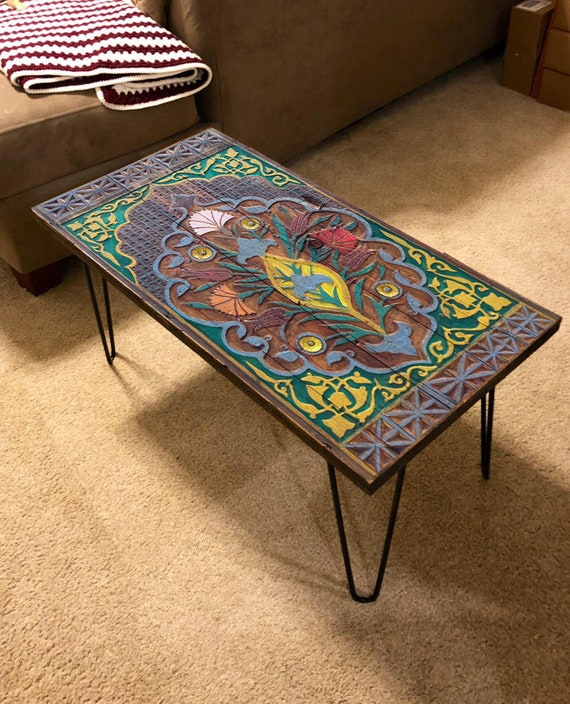The image depicts a small, heavily ornamented table situated in a well-lit indoor setting. The rectangular table features intricately bent, dark metallic legs that culminate in a curved flat spot at the bottom, giving it a stable yet delicate appearance. Each leg is thin and appears to be made of black wire, bent into a V-type shape to support the table at each corner, with three legs clearly visible from the bottom right corner perspective. 

The table's surface is richly decorated, designed to look like dark brown painted wood adorned with elaborate floral carvings. These decorations include a main central feature resembling a rosebud with various flowers extending from it, showcasing petals in hues of yellow, blue, green, red, orange, and white. Surrounding this central design, there are detailed blue and gold floral trims running along the edges, enhancing the table's ornamental appearance with sharp, wavy, and pointy designs.

The table sits atop a thick, light brown carpet, and in the background, the edge of a brown or tan sofa is visible, accompanied by a red and white striped throw draped at its foot. The image is brightly illuminated, suggesting it was taken indoors with ample natural or artificial lighting, casting soft shadows onto the carpet.